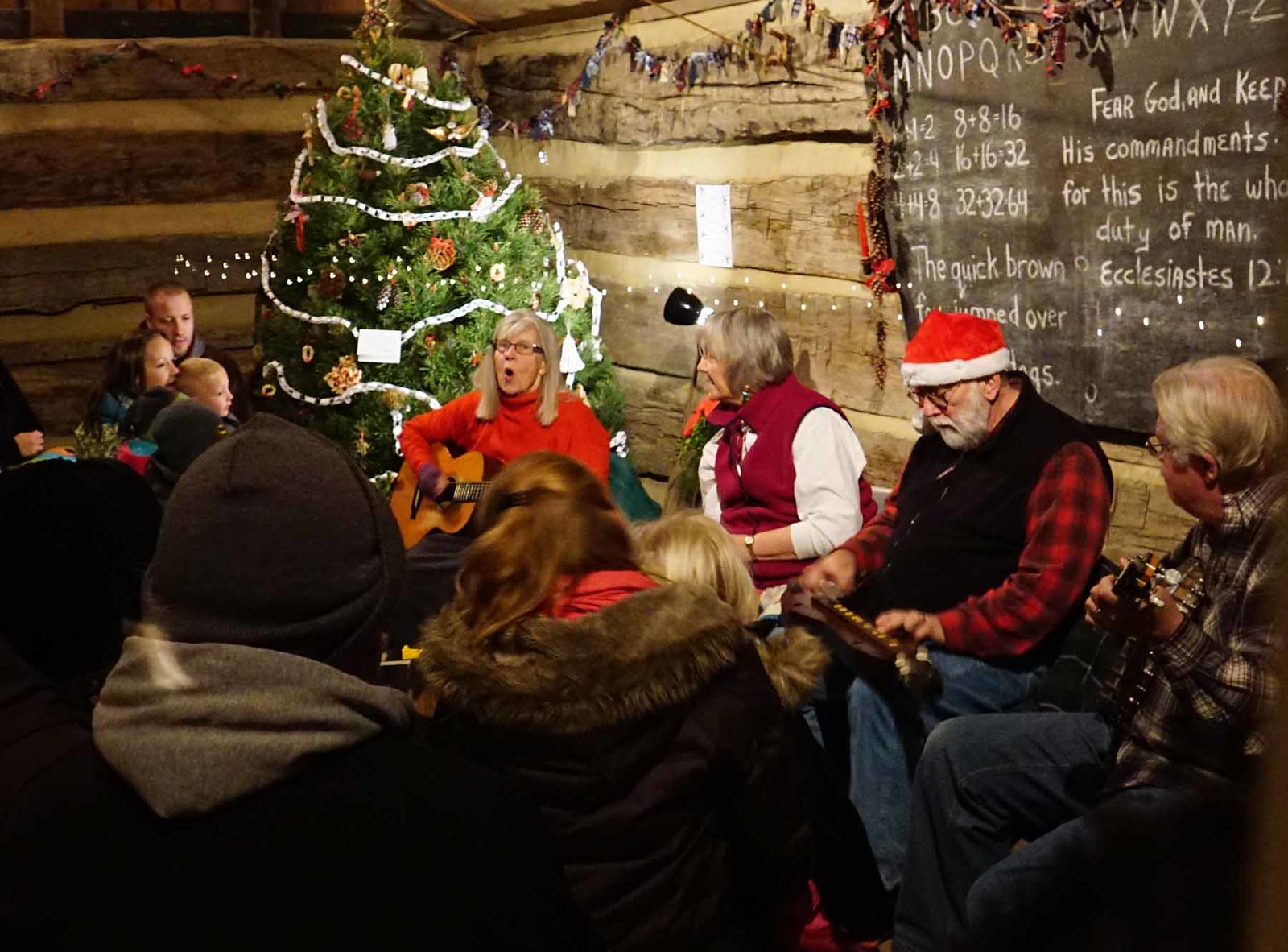In the cozy interior of a log cabin, a warmly decorated Christmas scene unfolds. A brightly adorned Christmas tree, wrapped in tinsel, stands tall in the corner where two wooden walls meet. Above the scene, a blackboard displays handwritten chalk letters reading “MNOPQRSTUVWXYZ” and a partial verse: “Fear God and keep his commandments, for this is the whole duty of man.”

The centerpiece of the gathering is a small group of musicians seated along the log wall. At the forefront is a woman in a red sweater, strumming a guitar and singing. To her right, three other musicians add to the festive atmosphere: a woman in a red vest over a white shirt, a man in a gray and black plaid shirt with white hair playing another guitar, and a man in a red and black checked shirt, blue jeans, and a black vest, distinguished by his red and white Santa Claus hat, who has a keyboard resting on his lap. 

In the cozy background, additional holiday decorations adorn the walls, contributing to the festive ambiance. Watching the performance, several people and children are visible in the lower left corner of the image, completely captivated by the musical celebration.